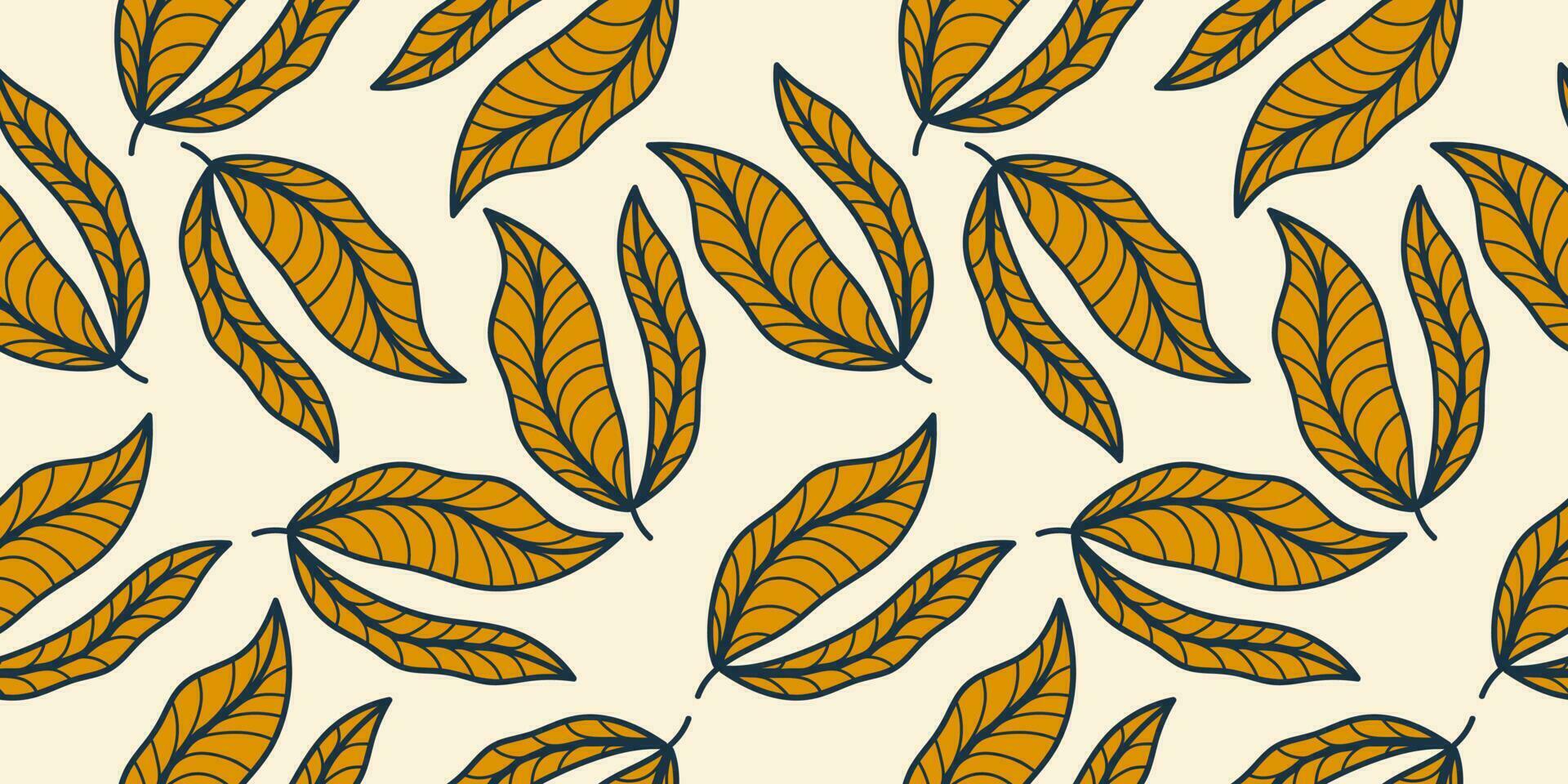This image is a cartoon or computer-generated graphic featuring a repeating pattern of paired leaves. Each pair consists of one slightly larger, wider leaf and one slightly slimmer, narrower leaf, both tapering to a point and connected by a short stem. The leaves, colored in a yellowish to mustard gold hue, exhibit detailed textures with visible veins. Set against a slightly off-white background, approximately 10 to 12 pairs are distributed throughout the image in a seemingly random, non-uniform rotation. The pattern, evoking a light and cheerful autumnal feel, resembles designs suited for wallpaper, t-shirts, blankets, or scrapbooking.